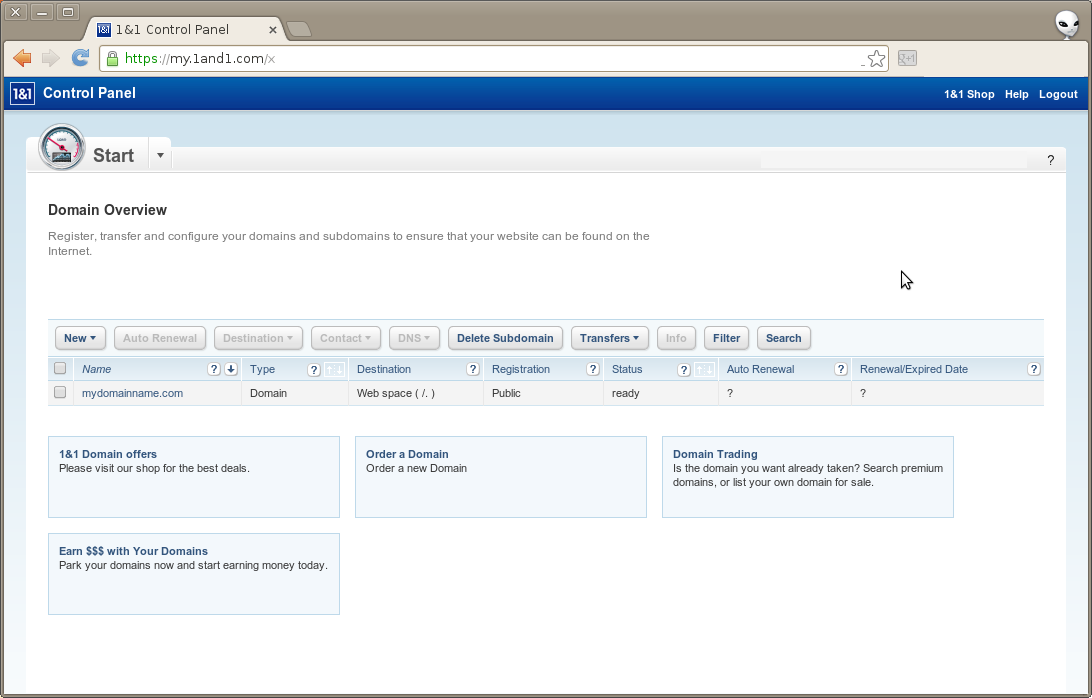The image depicts an old-style message screen providing particulars about a domain overview. At the top of the website is a gray rectangular bar stretching across the entire width of the page. Inside this bar are small white icons, and on the extreme right side is a small image of an alien face - a peculiar head with large black eyes, adding an intriguing touch.

Directly below the gray bar, there is a window tab area with a gray font that reads "One-on-One Control Panel." This section includes several functional icons: a search bar, a refresh key, a back key, and a forward key. Additionally, there is an option to star the website for future reference. 

Beneath this, a blue rectangle spans the width of the website, displaying "One-on-One Control Panel" in white font. To the right of this blue bar are links labeled "One-on-One Shop," "Help," and "Log Out."

Finally, the detailed overview of the domain begins below these navigational elements, providing a structured and comprehensive interface for users to manage their domain preferences and settings.